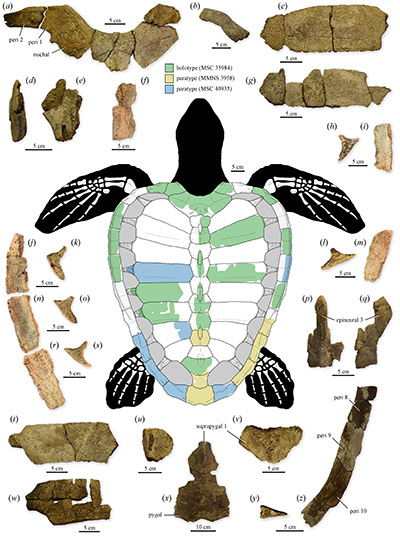The image is a detailed drawing of a sea turtle against a white background. The turtle is positioned vertically with its nose pointing towards the top of the image. It features a black head and black flippers with skeletal structures showing through them. The turtle's shell is a mixture of white, green, and gray colors. Surrounding the turtle are various diagrams and actual bone structures, each annotated and labeled meticulously.

To the left corner of the image, there are brown-colored bones and various markings. These bones are segmented and annotated with measurements, some labeled as 4 or 5 centimeters. There are multiple legends with small, difficult-to-read print, some of which include terms like "MSC35934," "paratype," and "horotype,” with alphanumeric codes like "M-M-N-5-3-9-5-9-3."

The annotations provide a detailed legend for each labeled part, going from letters A to Z, identifying specific bones or rock-like structures with corresponding measurements. For example, H is noted as an arrowhead at 5 centimeters, J and K are brown bones at 5 centimeters, and U is a D-shaped bone at 5 centimeters.

The image combines colored and realistic representations of the turtle’s anatomy with an educational layout, showing both the artistic and scientific interpretations of the turtle's skeletal structure and how each bone fits into the animal's anatomy.